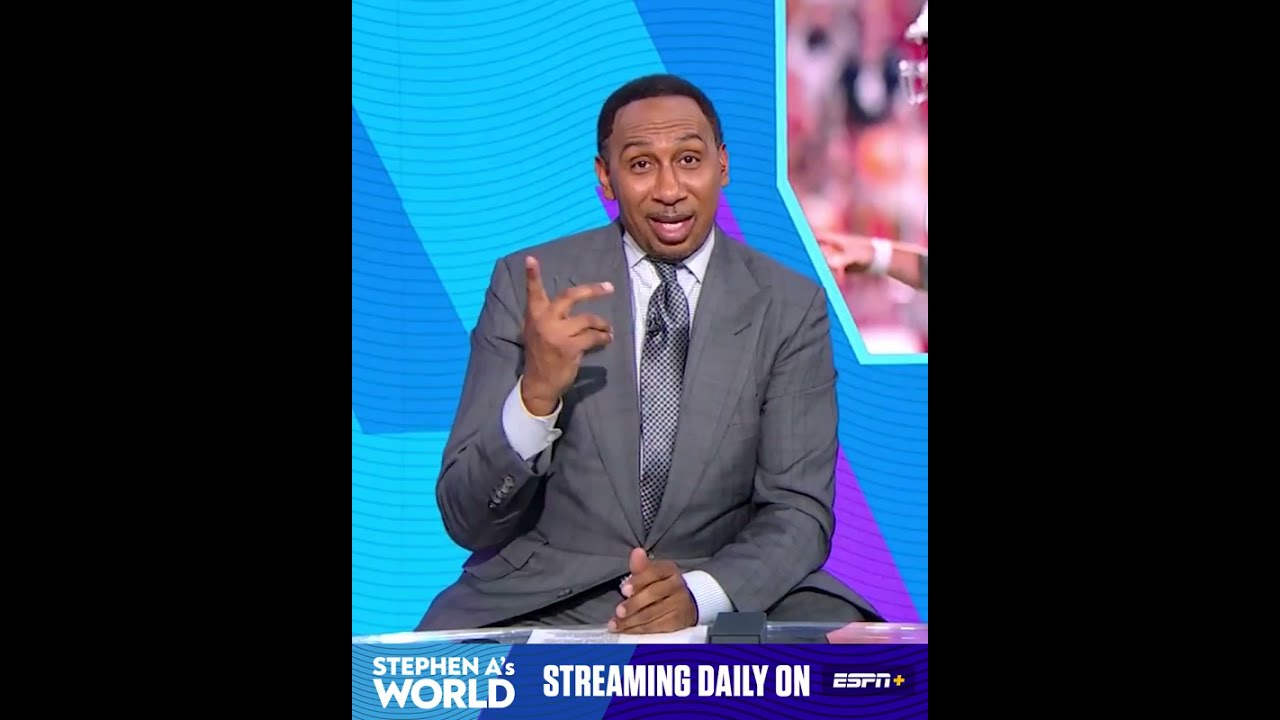The image features a black man in the center, wearing a well-tailored gray suit, a white shirt, and a silver tie. He is on a television show, facing the camera with an animated, questioning expression. His left hand rests on his leg, while his right hand is bent upwards as if gesticulating and speaking. The backdrop behind him showcases a vibrant mix of turquoise, purple, and blue streaks. Beneath him, a banner displays in white letters: "Stephen A's World," followed by "Streaming daily on ESPN." The image is framed with black bands on the left and right edges. The scene appears to be a screenshot from a streaming service, likely showcasing a sports announcement or discussion.